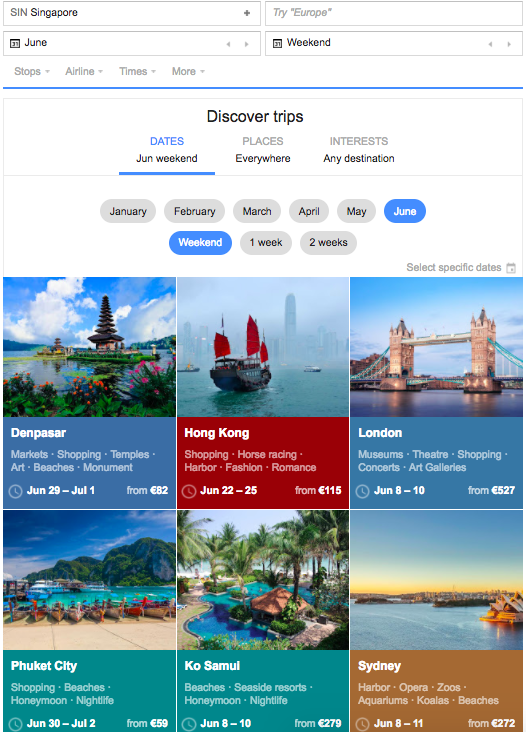Top left of the image displays the header "SIN Singapore" along with the date "June." On the left side, another header reads "Try Europe" with the date labeled as "weekend." Below these headings, a series of dropdown menus are situated, including "Shop," "Stops," "Airline," "Times," and "More," each highlighted with a blue underline.

At the center of the image, the prominent text "Discover Trips" is listed in black. Additionally, three tabs labeled "Date," "Places," and "Interest" accompany the text. The "Date" tab is underlined and highlighted in blue, with options for selecting months displayed below it in grey boxes ranging from "January" to "June," with "June" specifically highlighted in blue. Additional options include choices for the trip duration: "Weekend," "One Week," or "Two Weeks," with "Weekend" highlighted in blue.

Central to the image, six pictures showcase various travel destinations:

1. **Denpasar, Bali**:
   - Themes: Market shopping, temples, arts, beaches, monument
   - Travel dates: June 29 to July 1
   - Starting price: From 82 euros

2. **Hong Kong**:
   - Themes: Shopping, horse racing, harbor, fishing, romance
   - Travel dates: July 22 to 25
   - Starting price: From 115 euros

3. **London, UK**:
   - Themes: Museum, theatre, shopping, contests, art galleries
   - Travel dates: June 8 to June 10
   - Starting price: From 127 euros

4. **Phuket, Thailand**:
   - Themes: City shopping, beaches, honeymoon, nightlife
   - Travel dates: June 30 to July 2
   - Starting price: From 59 euros

5. **Kuala Lumpur, Malaysia**:
   - Themes: Beaches, seaside, resort, honeymoon, nightlife
   - Travel dates: June 8 to June 10
   - Starting price: From 279 euros

6. **Sydney, Australia**:
   - Themes: Harbour, opera, zoos, aquariums, koalas, beaches
   - Travel dates: June 8 to June 11
   - Starting price: From 272 euros

Each destination is vividly depicted with images highlighting their unique attractions.